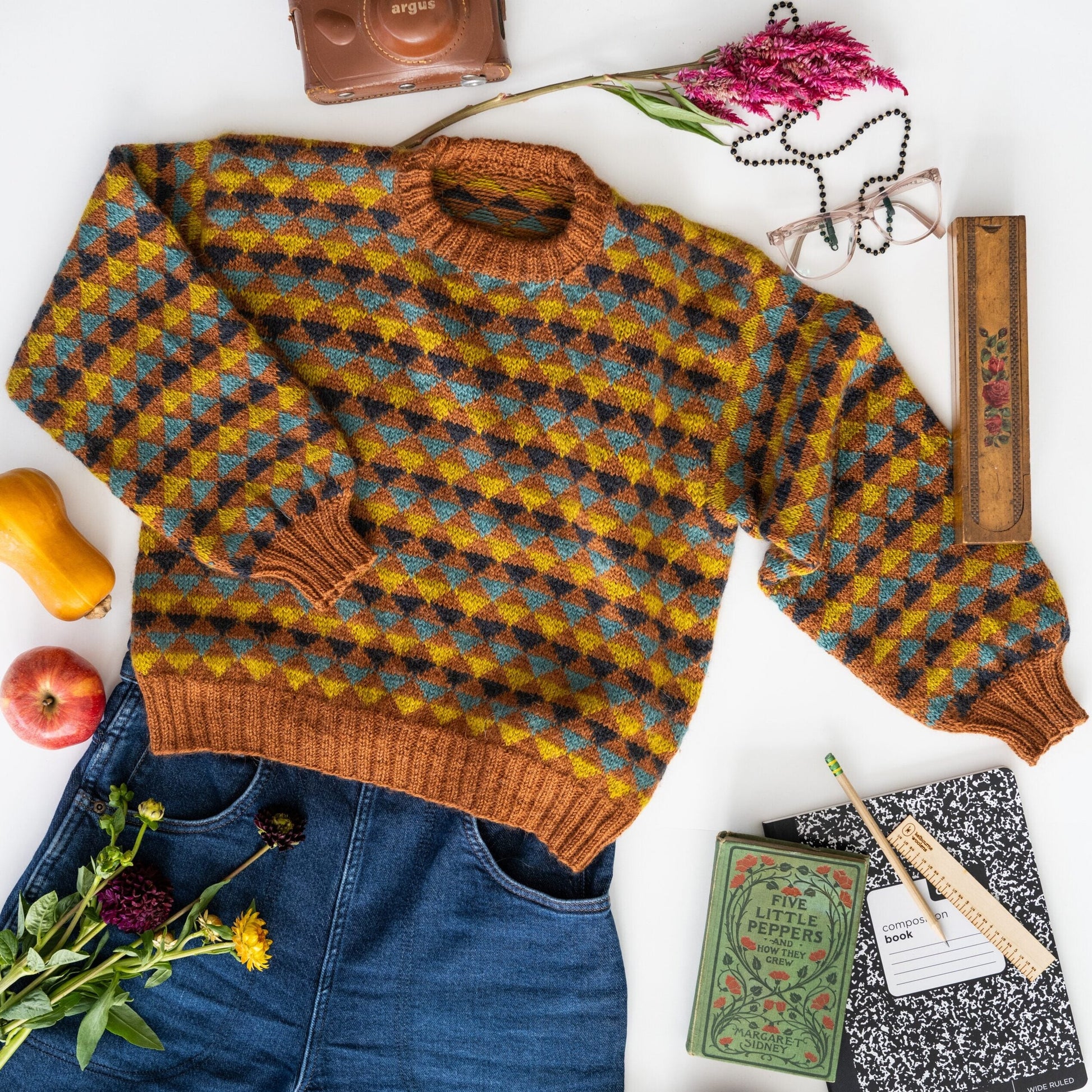The image showcases a meticulously arranged product shot on a white background, featuring various objects that suggest a back-to-school or autumn theme. The central item is a pullover sweater, adorned with a vibrant triangle print in colors of blue, green, yellow, and black, set against a honey-brown base. The sweater, complete with a brown crew neck, cuffs, and waist borders, is paired with dark blue jeans positioned directly beneath it.

To the left of the sweater, there's a squash and a red apple, adding a touch of seasonal produce. Nearby is a green book titled "Five Little Peppers" and a black and white marbled composition notebook, accompanied by a small wooden ruler and a brown pencil with a green aluminum band. On the bottom right of the image, additional yellow and dark maroon flowers can be seen.

Above the sweater, a variety of accessories are laid out. A small black beaded necklace, a pair of eyeglasses, and a brown camera case are positioned near a plant with hot pink, spiky-textured flowers on a brownish-green stem. This arrangement gives the image a cohesive, visually appealing composition, ideal for an advertisement or magazine layout.